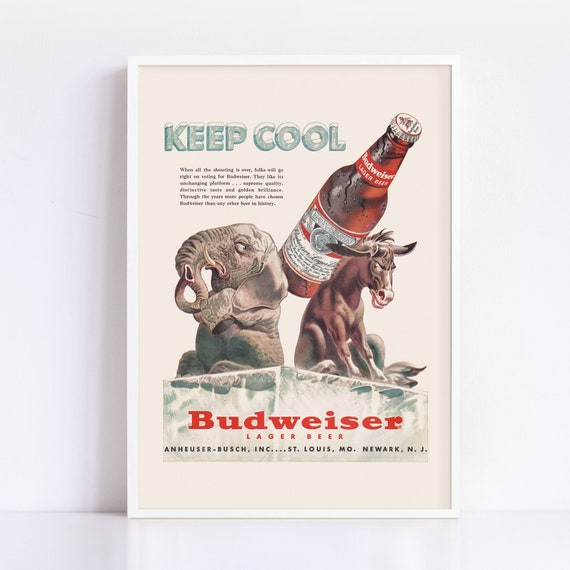In this vintage Budweiser advertisement, which is framed in white and set against an all-white backdrop, an elephant and a Clydesdale horse are sitting back-to-back atop a large ice cube. Both animals appear to be annoyed, casting side-eyes at each other. The Clydesdale has a cold-looking, condensation-covered bottle of Budweiser beer resting across its back. The ice cube prominently features the Budweiser logo in red, followed by the text "Lager Beer" and "Anheuser-Busch Inc., St. Louis, Missouri, Newark, New Jersey." Above the animals, the phrase "Keep Cool" is creatively displayed to look as though it's covered in ice and snow. There's additional, smaller text below the "Keep Cool" slogan that is not legible. The overall setting and design suggest a playful yet chilly atmosphere, highlighting the refreshing nature of the beer.